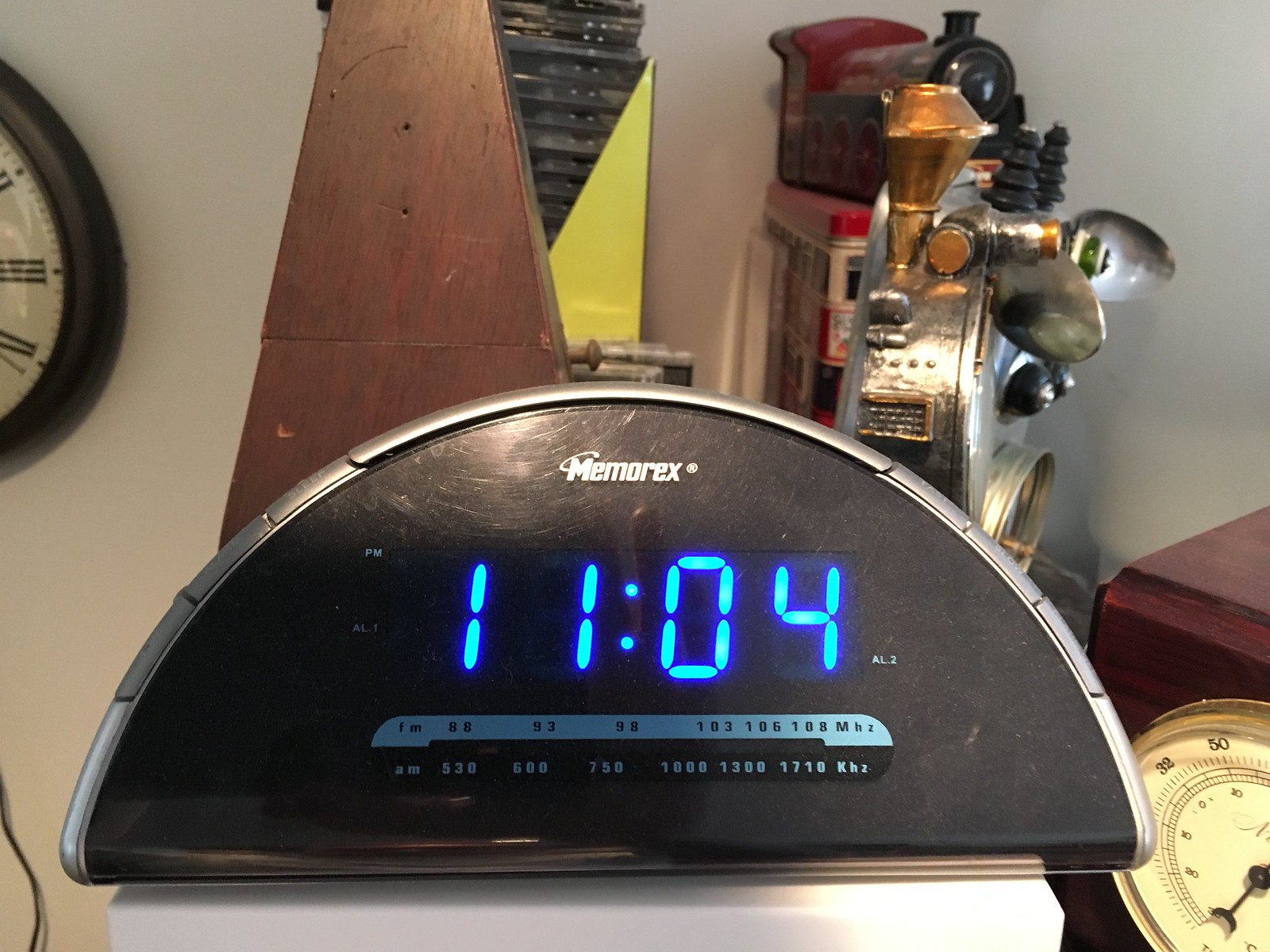This photograph showcases a vintage alarm clock with an integrated radio at the center, prominently displaying the brand name "Memorex" above a blue LED readout showing the time "11:04." The clock has a unique semicircular design, blending both modern digital and classic analog features. The radio frequencies are clearly labeled, with FM bands ranging from 88 to 108 MHz and AM bands from 530 to 1710 kHz, providing an insight into its versatile functionality.

Above and slightly to the left of the alarm clock, there is a wall clock partially visible, featuring Roman numerals that hint at an antique design. To the back of the main clock, a metronome stands quietly, suggesting a musical aspect to the collection of items. The background includes a few metallic objects, potentially components of a timepiece or scientific instruments, adding to the eclectic mix.

On the far right, there is an enigmatic chronometer, evoking the style of an artifact that belongs in a museum, further contributing to the old-world charm and historical intrigue of the scene. The arrangement of objects, with their varied functionalities and vintage aesthetics, paints a picture of a meticulously curated collection that captures the essence of timekeeping through the ages.